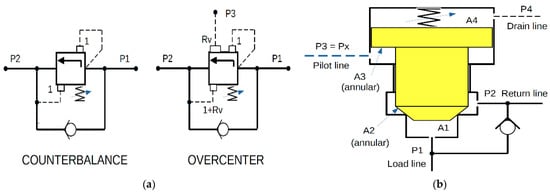The image features a complex technical diagram consisting of multiple interconnected components. On the left side, there are two smaller square diagrams labeled "A". The first square is labeled "Counterbalance," and the second is labeled "Over-center." Both of these diagrams have lines and arrows, some of which are dotted, indicating various directions and flows. To the right of these squares is a larger, more detailed diagram. This larger part is outlined in black and contains several dotted lines, but its central section is filled in with a yellow color characterized by a zigzag pattern at the top. Various parts of this diagram are labeled with technical terms including "Pilot Line," "Annular," "Return Line," "Drain Line," and "Load Line," as well as specific markings such as "P4," "P3," "A3," "P2," "A2," and "P1." The overall layout visually explains the relationships and functions of these components, focusing on hydraulic or pneumatic systems as suggested by the terminology.